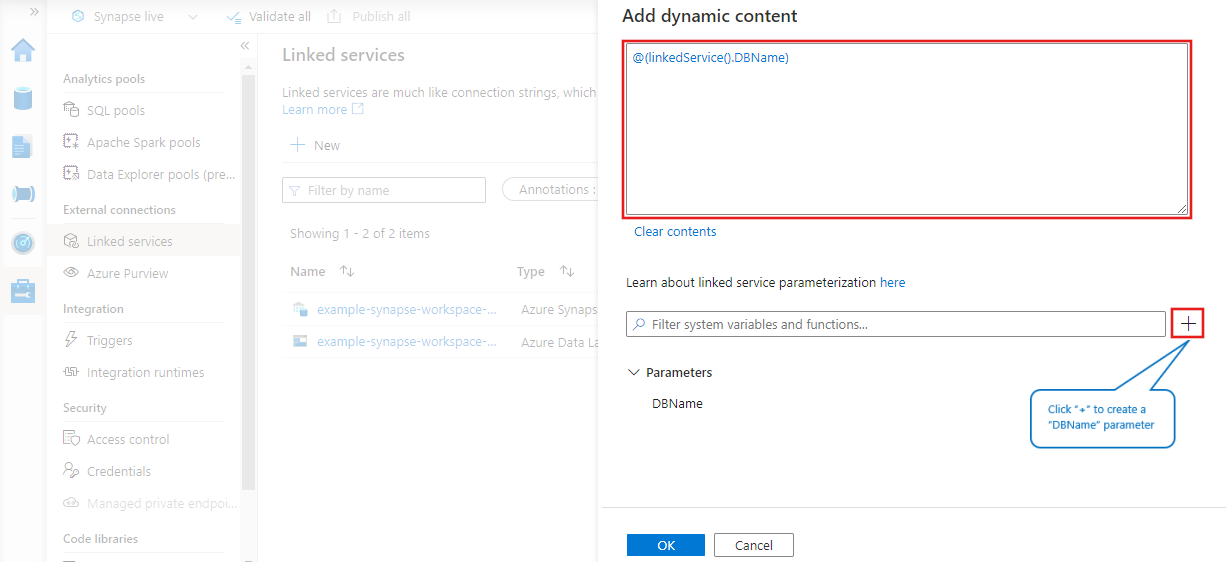The image portrays a backend interface of a web page setup, divided into three distinct panels. The two leftmost panels are grayed out, directing attention to the rightmost, prominent panel. At the top of this right panel, there is a header that reads "Add Dynamic Content," with a highlighted red box beneath it displaying "Add Linked Service (DB Name)." Below this box, the option "Clear Contents" is visible.

There is also a hyperlink labeled "Learn About Linked Service Parameterization Here," suggesting additional resources or documentation. Below this hyperlink, a search bar titled "Filter System Variables and Functions" is present, designed for searching specific variables or functions within the system.

A red-highlighted plus sign is positioned next to a section titled "Parameters," under which "DB Name" is listed. Adjacent to the plus sign, a thought bubble advises, "Click plus to create a DB name parameter." At the bottom of the interface, user action buttons labeled "OK" and "Cancel" are available, providing options to confirm or dismiss any changes made.

Overall, the image emphasizes the process of adding dynamic content to a web page via a linked service and highlights key interactive elements within the interface.